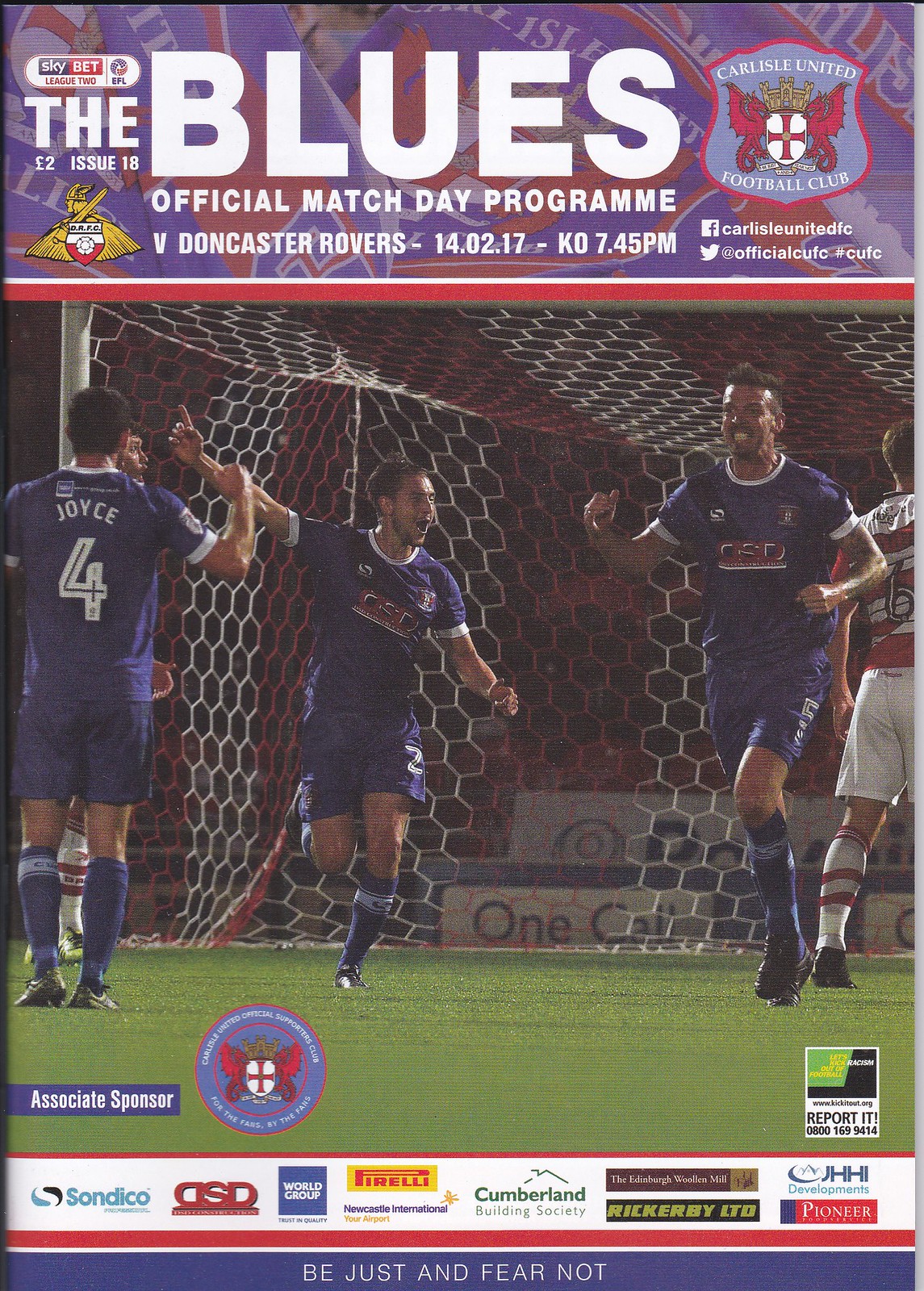The image is that of a vibrant and colorful magazine or program cover for a soccer match. At the top, it prominently announces "The Blues Official Match Day Program V Doncaster Rovers - 14.02.17 - KO 7:45 p.m.". This text is set against a backdrop of Carlisle United flags. To the right of this headline, the Carlisle United Football Club's regal logo is displayed, alongside social media links for Facebook (Carlisle United FC) and Twitter (@official CUFC, #CUFC). On the left, the Doncaster Rovers logo, featuring a Viking with a shield and sword, is visible. Below the headline, a dynamic photo captures three soccer players in blue uniforms celebrating a goal or victory. Two players, facing us, display exuberant expressions, while the third, seen from the back, is fist-pumping. Their shirts are marked with “GSD/CSD” and “Joyce” with the number 4. Additionally, a partially visible player in red and white, likely from the opposing team, appears on the field near a net with a red and white pattern. At the bottom, a blue bar lists sponsors such as Cumberland, San Dico, ASD World Group, Pirelli, and the Cumberland Building Society. A motivational text, “Be just and fear not,” adorns the bottom right.